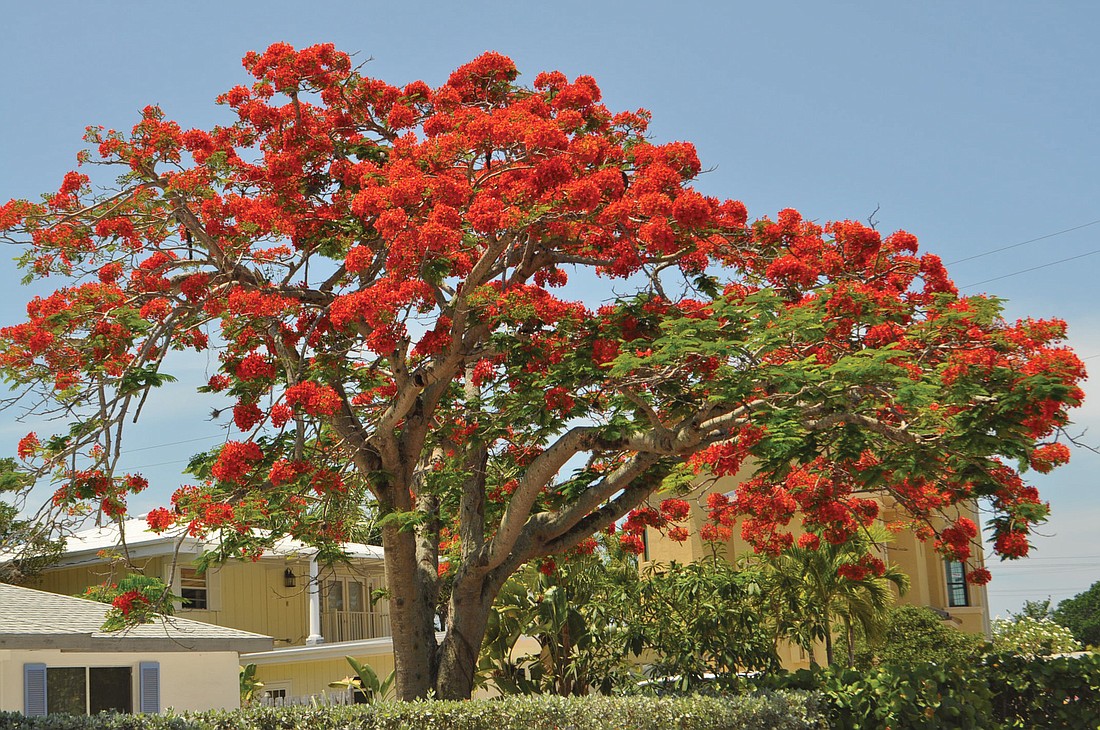The photo captures a vibrant scene centered around a large, unique tree with a tan trunk and sprawling limbs. The tree is adorned with fern-like green leaves and striking, spherical red blossoms, which are scattered abundantly across its branches. These red blooms stand out vividly against the greenery. At the base of the tree, there's a dense hedge or bush providing a lush, green foreground. The background features a bright blue sky and several buildings typical of a residential area. To the left of the tree is a two-story yellow house with a roof and windows, while slightly behind and to the right, another multi-story yellow house can be seen, partially obscured by the tree. Additionally, some electric power lines are visible around the tree, emphasizing the suburban setting.